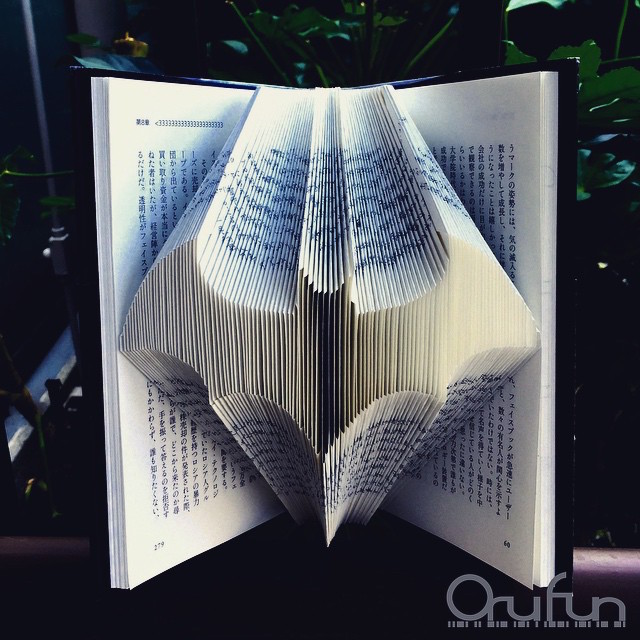This image displays an intricately crafted piece of book art. An open book, standing on its edges, features pages meticulously folded to create a three-dimensional Batman symbol, the iconic bat shape prominently emerging from its center. The pages, covered in Japanese or Chinese characters, suggest an Asian script that adds an exotic touch to the artwork. The book’s dark black binding contrasts sharply with its pages, emphasizing the elaborate folds. Notably, page numbers 279 and 60 are visible at the bottom corners on the left and right, respectively. A watermark or logo, reading "O-R-U-F-U-N," is subtly placed in the lower right-hand corner in light gray, with a dashed line below it. The background is primarily dark, with some shrubbery and a leafy plant slightly visible, creating a stark contrast that highlights the book and its artistic centerpiece. This captivating piece not only showcases the art of origami but also transforms an ordinary book into an extraordinary visual experience.